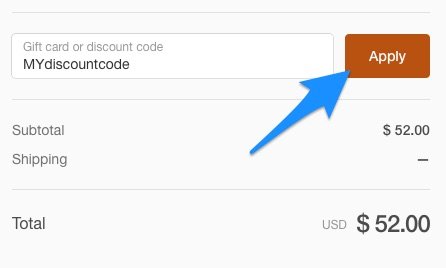A screenshot displays an online checkout page with a white box against a gray background. The box prompts for a "Gift card or discount code" and shows the entered code: "MYdiscountcode" (with "MY" in capital letters and "discountcode" in lowercase letters). A prominent blue arrow points towards an "Apply" button, which is rust-colored. Below the code input box, the order summary shows a subtotal of $52.00. The shipping cost is indicated by a dash, suggesting free shipping. The total amount due is also $52.00, marked in USD. It's unclear whether the blue arrow was added by the store or by the user. The applied discount code might be intended for a discount or free shipping. Despite the code, the subtotal and total remain identical at $52.00 USD.